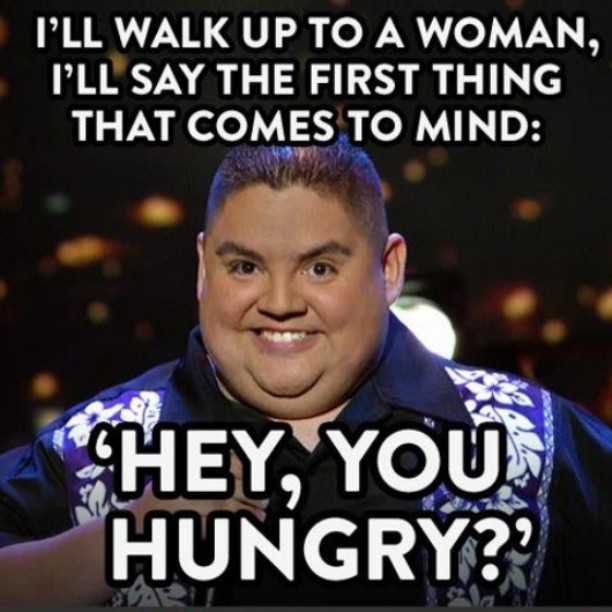The meme features a photograph of an obese man with light caramel-colored skin, short brown hair, and brown eyes. He has a broad, closed-lip smile that reveals his top row of teeth and showcases his double chin. The man is dressed in a navy blue collared shirt, adorned with a distinctive floral pattern on a purple band running along both sides of the shirt. In the background, there's a bright light between his ear and shoulder on the right side, contrasting with the dark, out-of-focus backdrop peppered with faint, round light spots. Captioned in all-capital, white sans-serif letters, the meme humorously reads: "I'LL WALK UP TO A WOMAN, I'LL SAY THE FIRST THING THAT COMES TO MIND, HEY, YOU HUNGRY?" The man's expression and attire suggest a self-deprecating joke, possibly alluding to his frequent thoughts of food, even in social situations with women, hinting that he might be a comedian mocking his own tendencies.